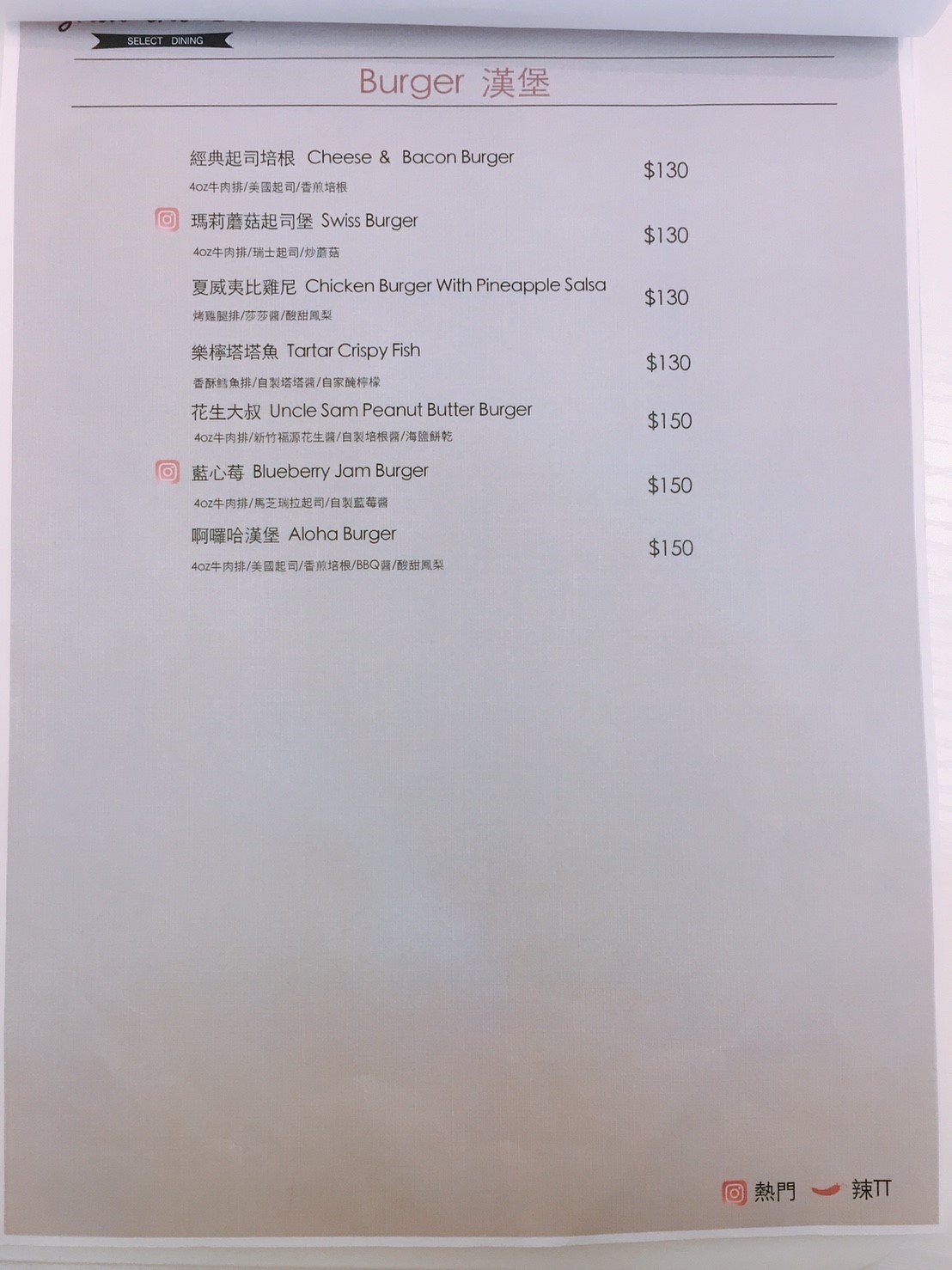The image features a menu item displayed on a white sheet of paper. At the top, the word "Burger" is prominently written in bold red letters in English, accompanied by the same word rendered in what appears to be either Chinese, Japanese, or Korean characters. Below this heading, the menu items are listed in black ink, starting with:

1. Cheese and Bacon Burger - $130
2. Swiss Burger - $130
3. Chicken Burger with Pineapple Salsa - $130
4. Tata Crispy Fish - $130
5. Uncle Sam Peanut Butter Burger - $150
6. Blueberry Jam Burger - $150
7. Aloha Burger - $150

Each item is neatly arranged in a vertical sequence, providing a diverse selection of unique and intriguing burger variations.